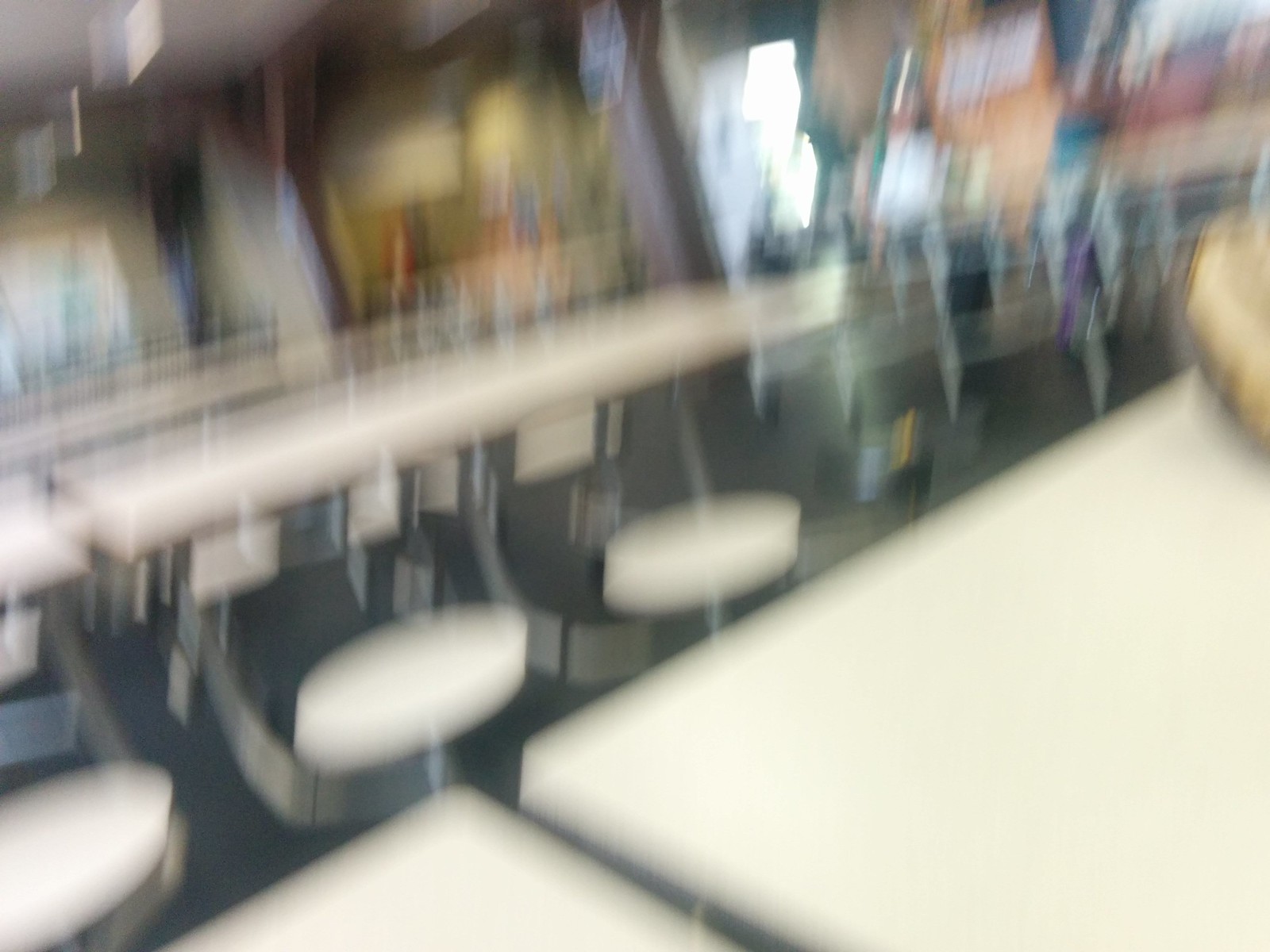A blurred motion shot taken inside what appears to be a school setting, possibly a classroom or cafeteria. The room features characteristic folding tables with attached white stools, typical of school furniture designed to accommodate eight to ten individuals. Despite the lack of clarity, the vivid colors in the room hint at an educational environment, though specific items on the walls and the presence of individuals are indiscernible.